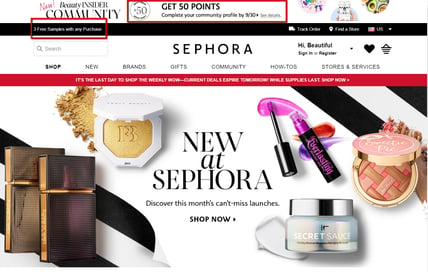The image depicts a screenshot of a website, specifically Sephora's. The screenshot is about 30-50% wider than it is tall. The background of the site is predominantly white. 

In the upper left corner, there is a logo or text that reads "Insider Community," although the details are somewhat difficult to discern due to the image's small size. Moving right, there is a circular icon featuring the number "50," surrounded by unreadable text. Adjacent to this icon, in bold text, it states "Get 50 points," followed by smaller text that says, "Complete your community profile by 9/30, see details."

Further right, there appear to be three indistinct objects, possibly jewelry. Below these elements is a menu bar with a black background and white text. The only legible part of this text is the phrase "any purchase," framed by a red box. This red box treatment is also applied around the "Get 50 points" text and the circular "50" icon.

Centrally located below the menu bar is the Sephora logo. To the left of the logo, there is a search bar, and to the right, welcoming text that says, "Hi beautiful."